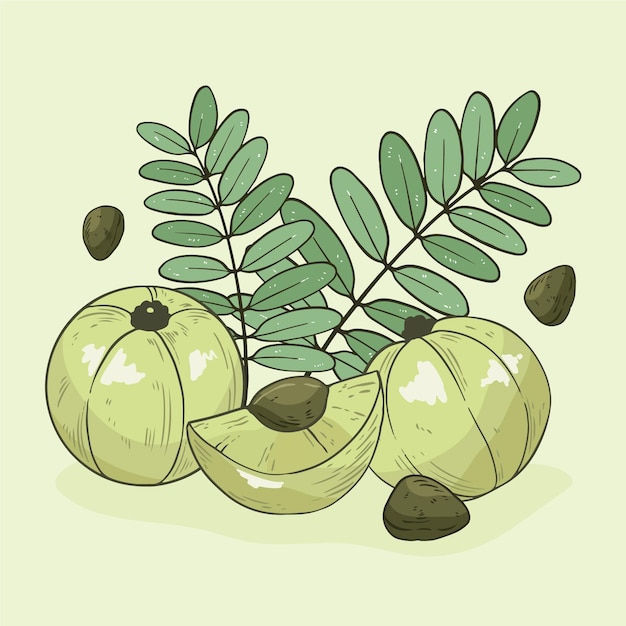The illustration depicts a collection of fruits and leaves in a neutral palette dominated by green hues. At the center, there are two whole fruits and one sliced open to reveal a dark brown stone or seed, alongside three additional separate stones. The fruit, which resembles a small pumpkin or an unidentified exotic variety, is light greenish-yellow with white highlights and about the size of a fist or slightly larger. The backdrop features two branches adorned with small, oval, sage-colored leaves and a very light beige background tinged with a touch of green, layering the scene with a serene and delicate ambiance.